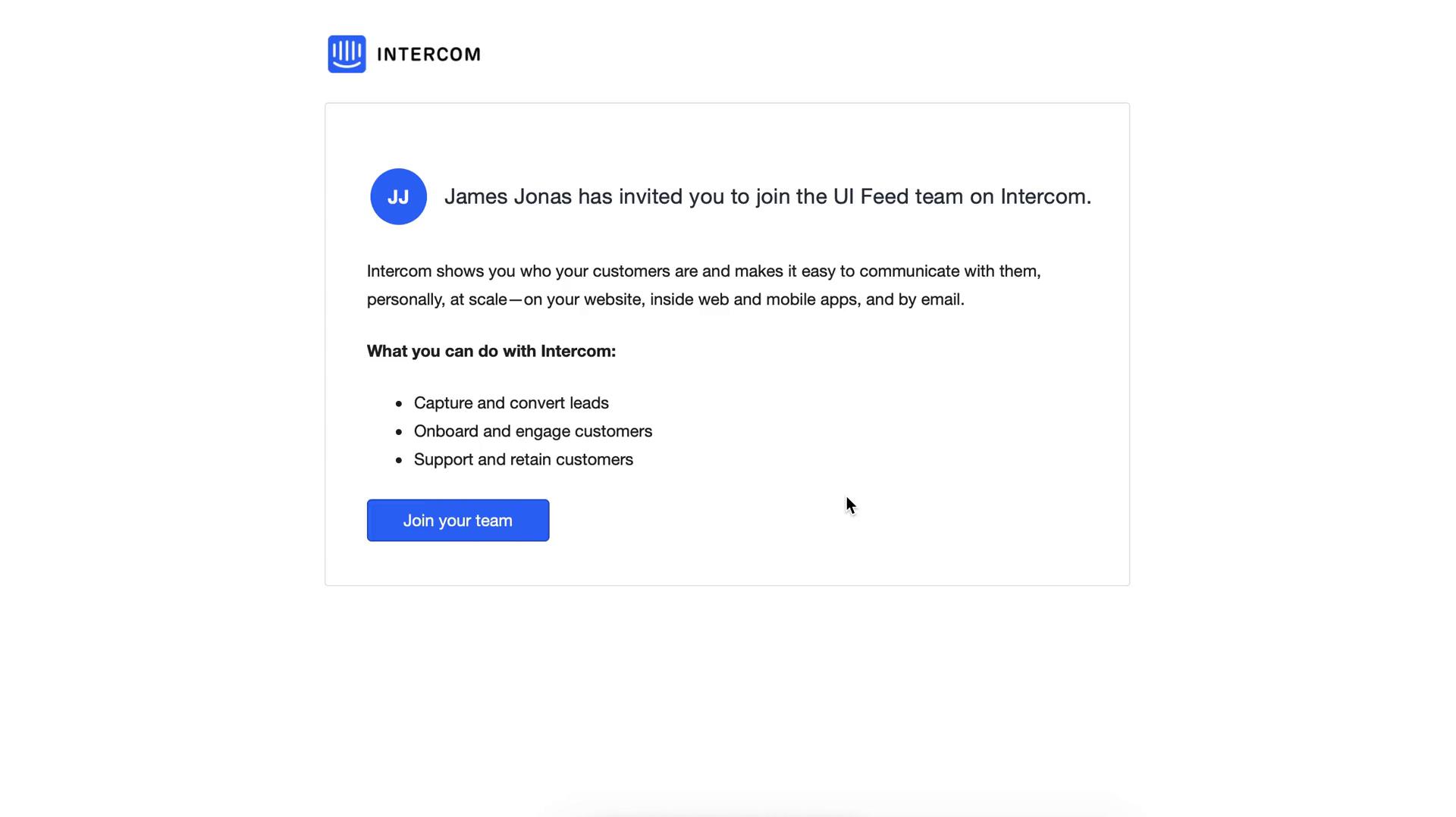A screenshot of the Intercom interface, likely a chat program, is depicted, showcasing various elements in detail. In the upper left corner, the Intercom logo is visible—comprised of a blue icon featuring a side-lying parenthesis at the bottom and a series of vertical lines above it—accompanied by the text "Intercom." Below the logo, there is a box with a faint black outline. Within this box, a circular blue icon with the initials "JJ" represents James Jonas, who has invited the user to join the UI Feed team on Intercom. A message explains that Intercom helps identify customers and facilitates personal-scale communication through a variety of platforms, including websites, web and mobile apps, and email. Additional information highlights Intercom’s capabilities, such as capturing and converting leads, onboarding and engaging customers, and supporting and retaining customers. A prominent blue button labeled "Join your team" is positioned at the bottom of the box, inviting the user to participate. This depiction suggests that Intercom functions as a Customer Relationship Management (CRM) system.